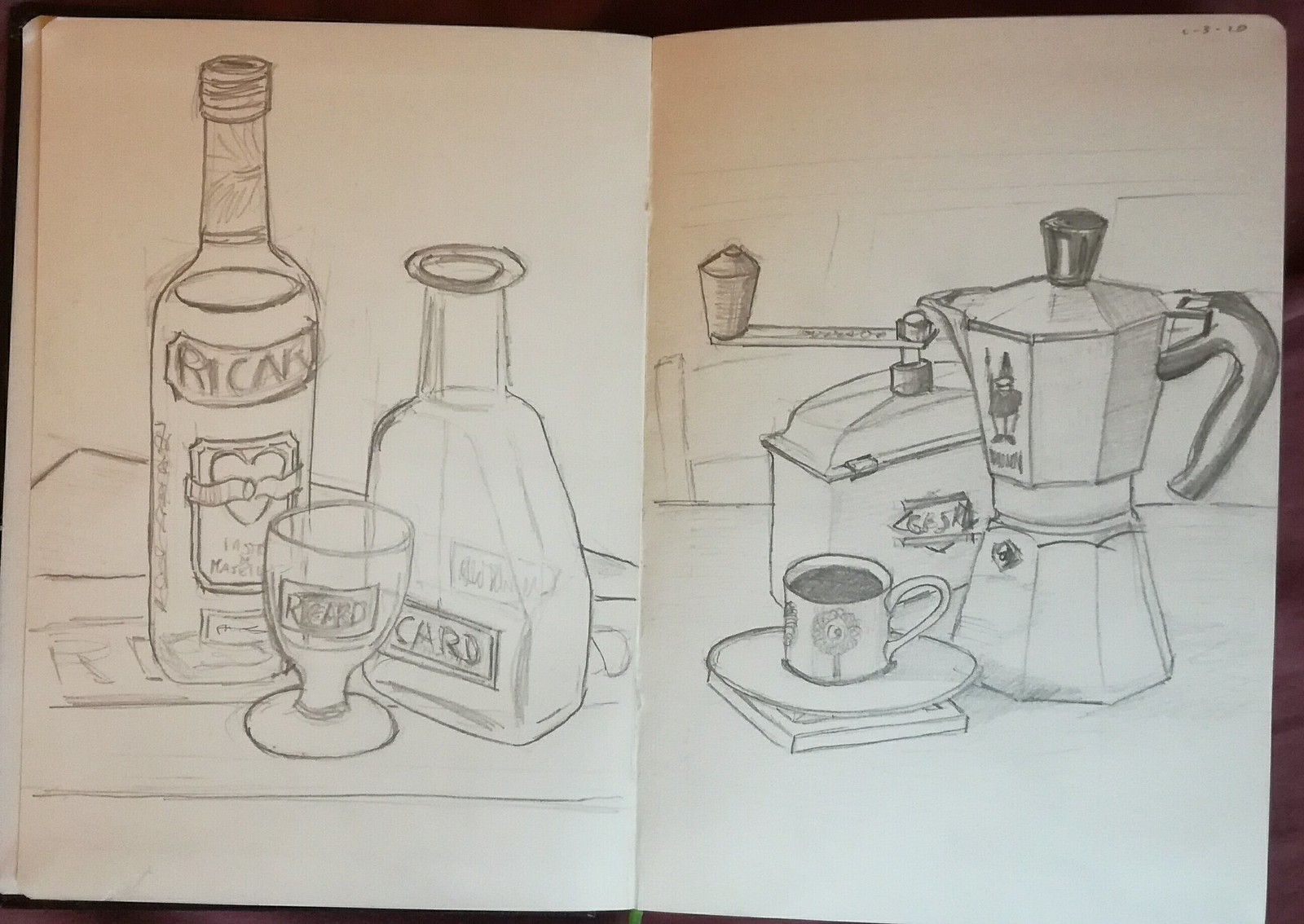In the image, set against a dark background, an open notebook is prominently displayed at the center, folded along its middle. On the left page, detailed pencil sketches capture a large bottle labeled "Eureka." The label features a square, within which is a heart embellished with a ribbon, inscribed with text, and another smaller square positioned at the bottom. The scene includes a cup labeled "Ricard," along with a wider bottle also marked "Ricard," which appears to be empty.

To the right side, a French pot, adorned with a distinctive gnome label, is depicted with a black handle and a unique top spout resembling a shaker. Nearby, there seems to be a jar of sugar or potentially a coffee grinder.

Additionally, a cup of brewed coffee is placed thoughtfully with delicate pencil flourishes on its side, resting on a dish set atop a coaster.